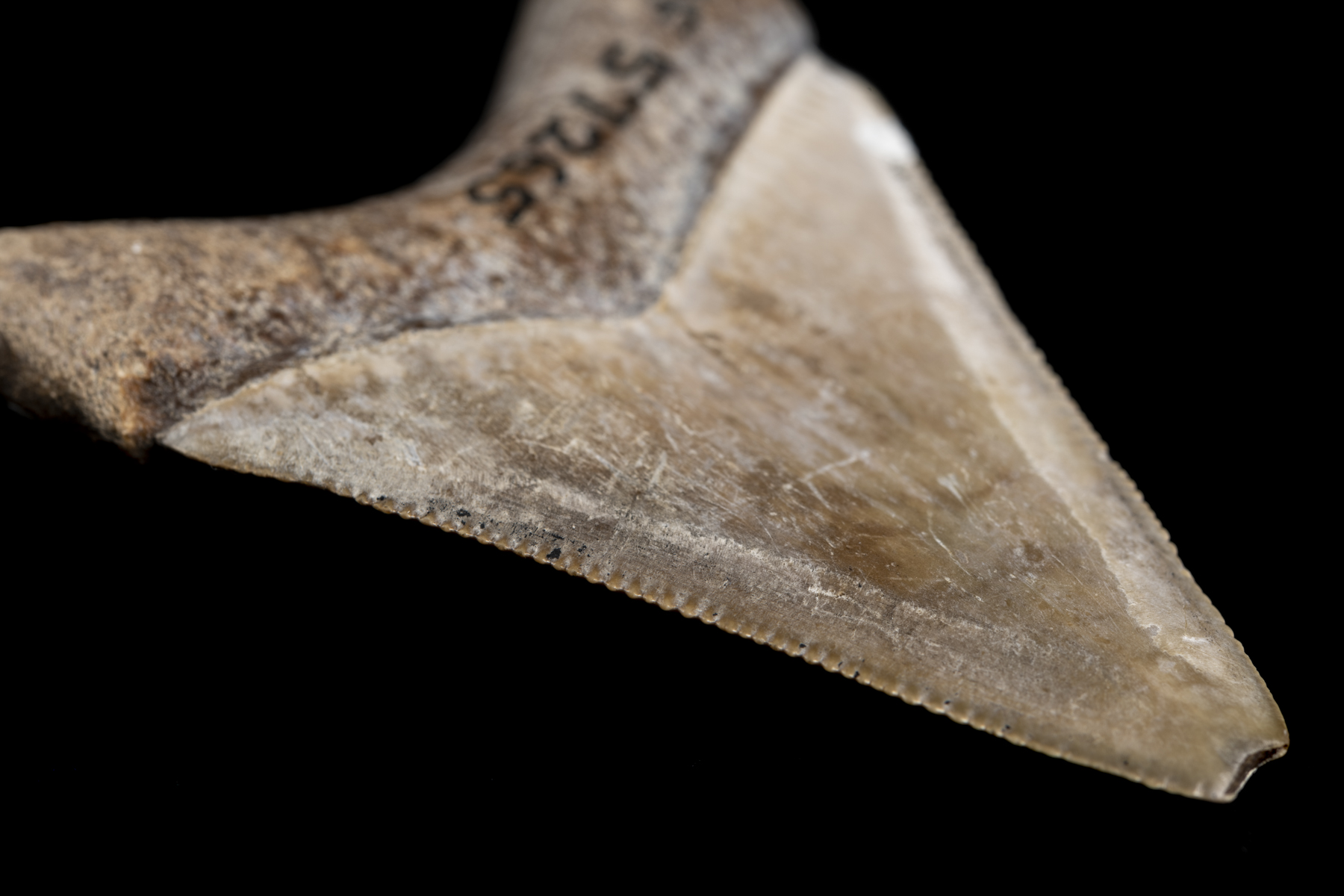The image features a close-up, detailed photograph of an artifact-like object that resembles a flint arrowhead or possibly a shark tooth. The object is predominantly triangular in shape with a distinct curved edge and is centered against a pitch-black background, emphasizing its form. The coloration of the piece is a mix of beige, gray, and brown hues, suggesting it might have crust and rust, indicative of age and wear. Toward the upper right part of the object, discernible lettering reads "SYLIS" or the numbers "57265," though part of these inscriptions might be cut off or upside down, making definitive reading challenging. The tip of the triangular object appears to be broken off, adding to its ancient, weathered look.